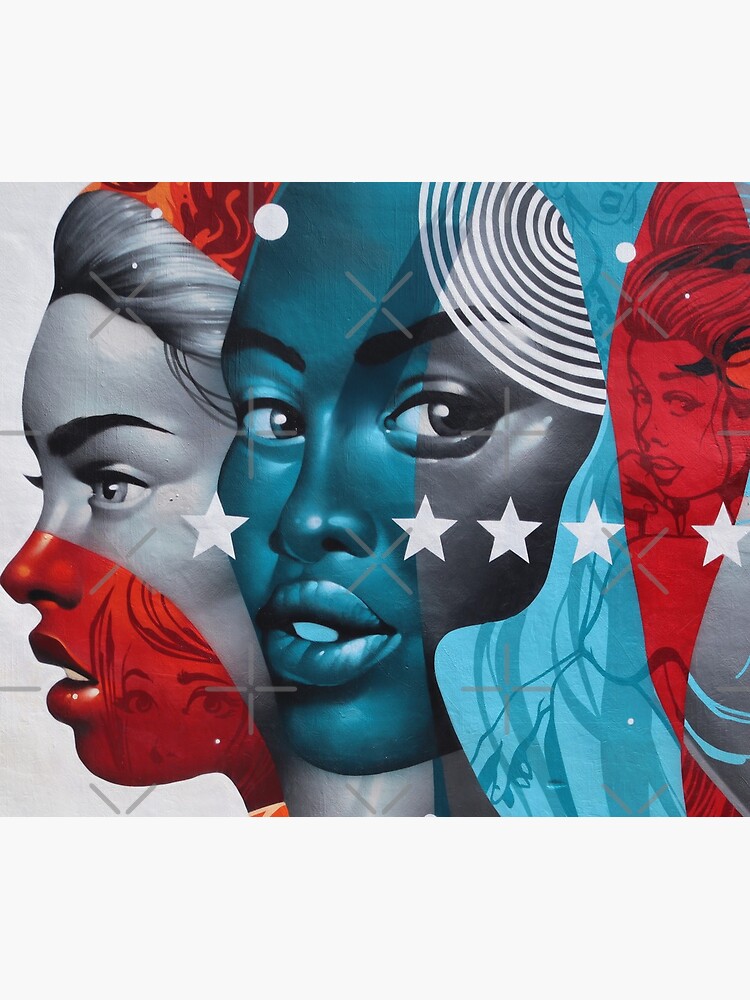The square image, centrally placed with thick light gray borders on the top and bottom, features a dynamic and colorful drawing of multiple human faces, stylized like comic book characters. Starting from the left, a woman with light-colored skin gazes leftward, her serious expression marked by a dark eyebrow and parted lips. The lower half of her face, from mid-nose down, is shaded red, contrasting sharply against the gray background that resembles a brick wall.

To the right, a woman with dark skin faces forward, her visage split into a blue and dark gray pattern. Her eyes, fully visible, convey a direct look. Decorating the blue side of her face, a white and gray spiral pattern winds intricately. White stars are positioned near her nose: one on the left and four on the right.

On the far right, a red and blue outline forms the profile of another woman looking over her shoulder. Her hair, drawn up elegantly, complements the red shading of her image. White stars and dots intersperse the drawing, adding an element of whimsy and depth to the composition.